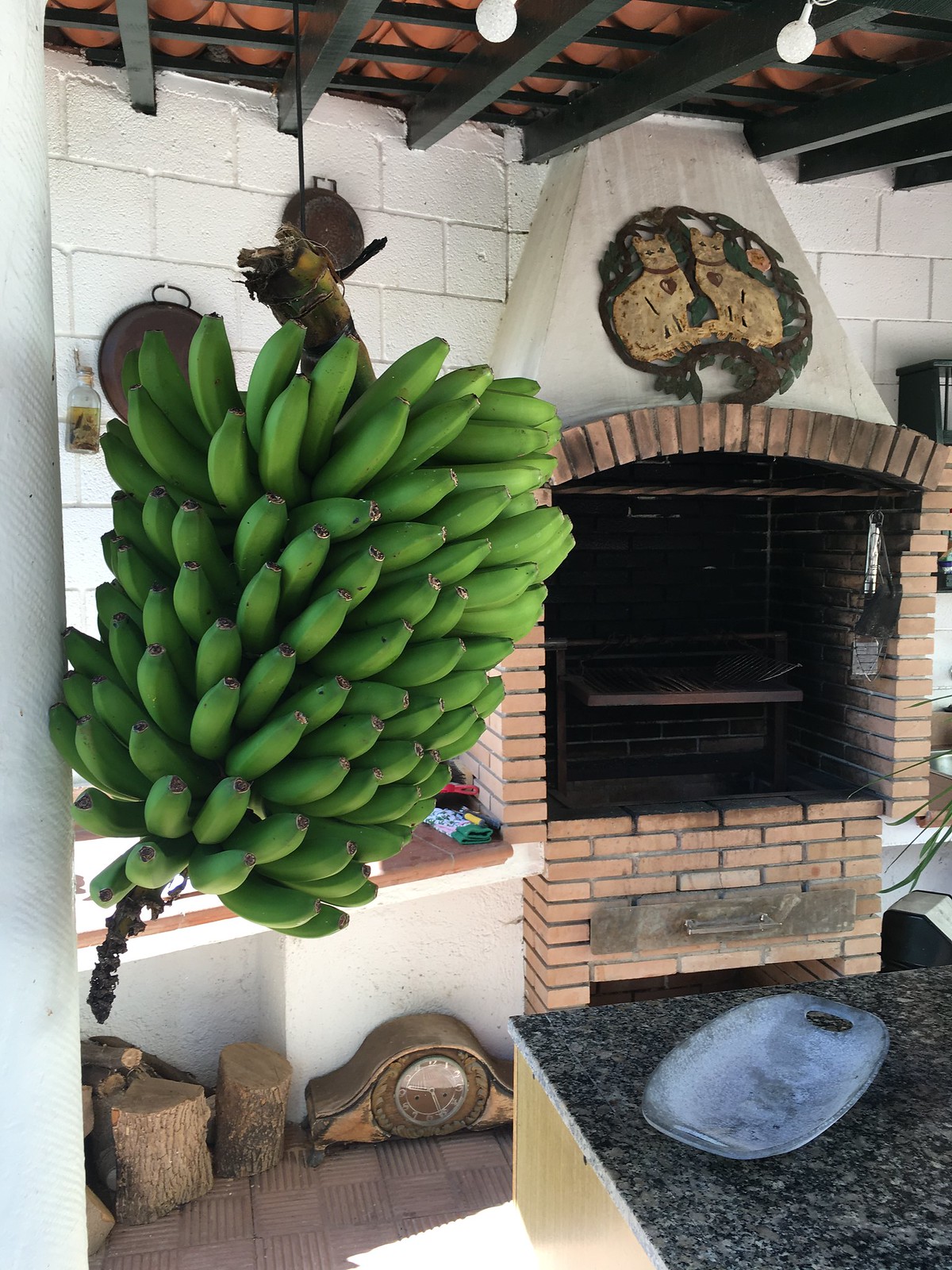The image depicts a wall oven built into a brick recess, crowned by a large flume with a decorative figurine featuring two tan cats with collars and heart pendants. A small counter juts out from the left side of the wall, where a metal tray sits atop a dark tabletop. Below the counter, a small clock rests on the floor, adjacent to neatly chopped logs. A lush banana bunch, dark green in color and apparently unripe, hangs by its stem from a greenery tree, indicating it's either part of an indoor setting with an outdoor vibe or vice versa. Overhead, several white light bulbs illuminate the scene.